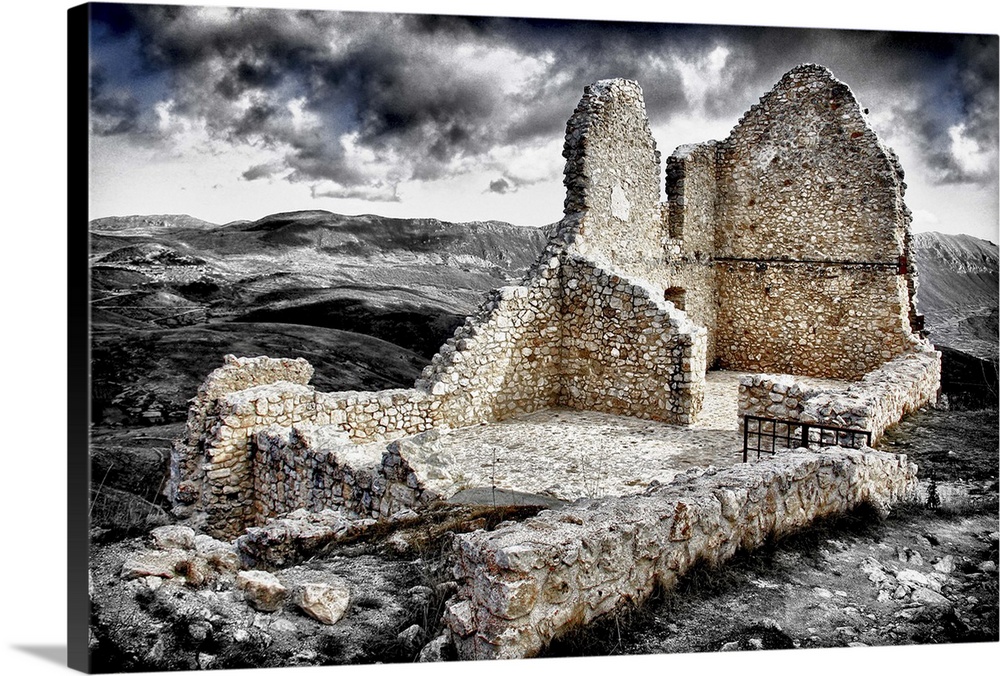In this striking product photograph, the canvas print is set against a flawless, featureless white background, creating the illusion that it is floating in an empty white void. The canvas edge, visible in the image, is black, accentuating the artwork's presentation. The photograph captures an evocative ruin scene, dramatically edited to highlight the ruin in full color against a stark black and white landscape, sky, and surrounding area. The ruin itself, constructed from large stone blocks in shades of brown, gray, and white, possesses a haunting, ancient quality. Most of the structure has crumbled, leaving only the back corner and foundation intact. The ruin features windows, a doorway, and a black metal railing at the front entryway. Dark, ominous clouds dominate the sky, lending a sense of foreboding to the composition, and the rocky, charcoal gray hills in the background further enhance the dramatic and eerie atmosphere.